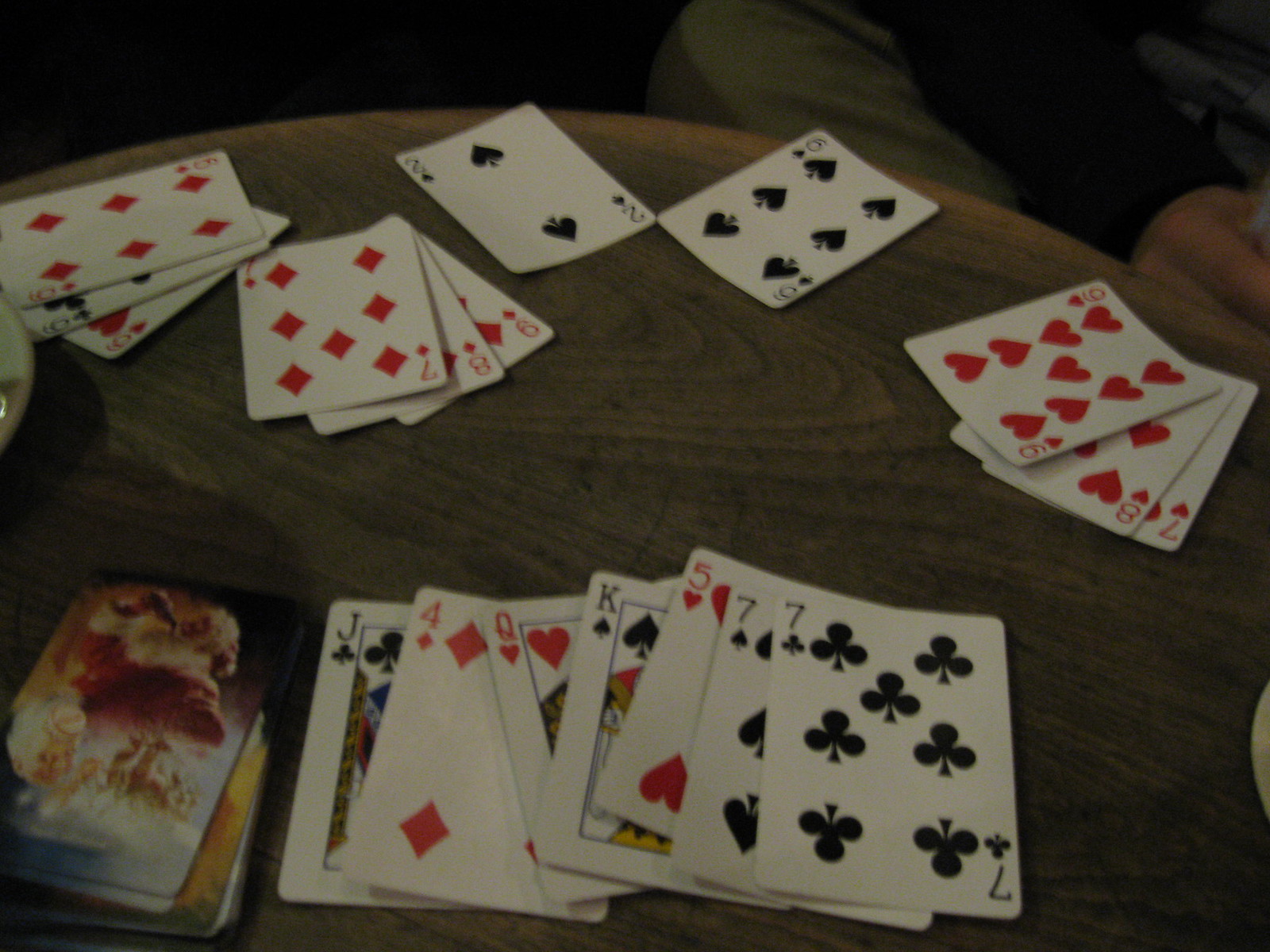In this dimly lit color photograph with a warm brown overlay, we see several neat stacks of playing cards spread out on a round wooden table. The cards are all face-up, allowing us to clearly see the details of each card. The stack closest to the camera consists of seven cards: a jack of clubs, a four of diamonds, a queen of hearts, a king of spades, a five of hearts, a seven of spades, and a seven of clubs. 

Around the edge of the table, there are more stacks, seemingly placed where people had been sitting, suggesting a recently interrupted game. In addition to these stacks, an organized deck of cards lies to the side, its colorful back design partly obscured, hinting at whimsical imagery that could be a cloud or perhaps reindeer. 

A plate or dish, partly visible among the cards, adds a casual touch to the scene, reinforcing the impression of a relaxed, social atmosphere. The combination of the scattered, face-up playing cards and the household dishware creates a vivid snapshot of an engaging moment among friends or family.